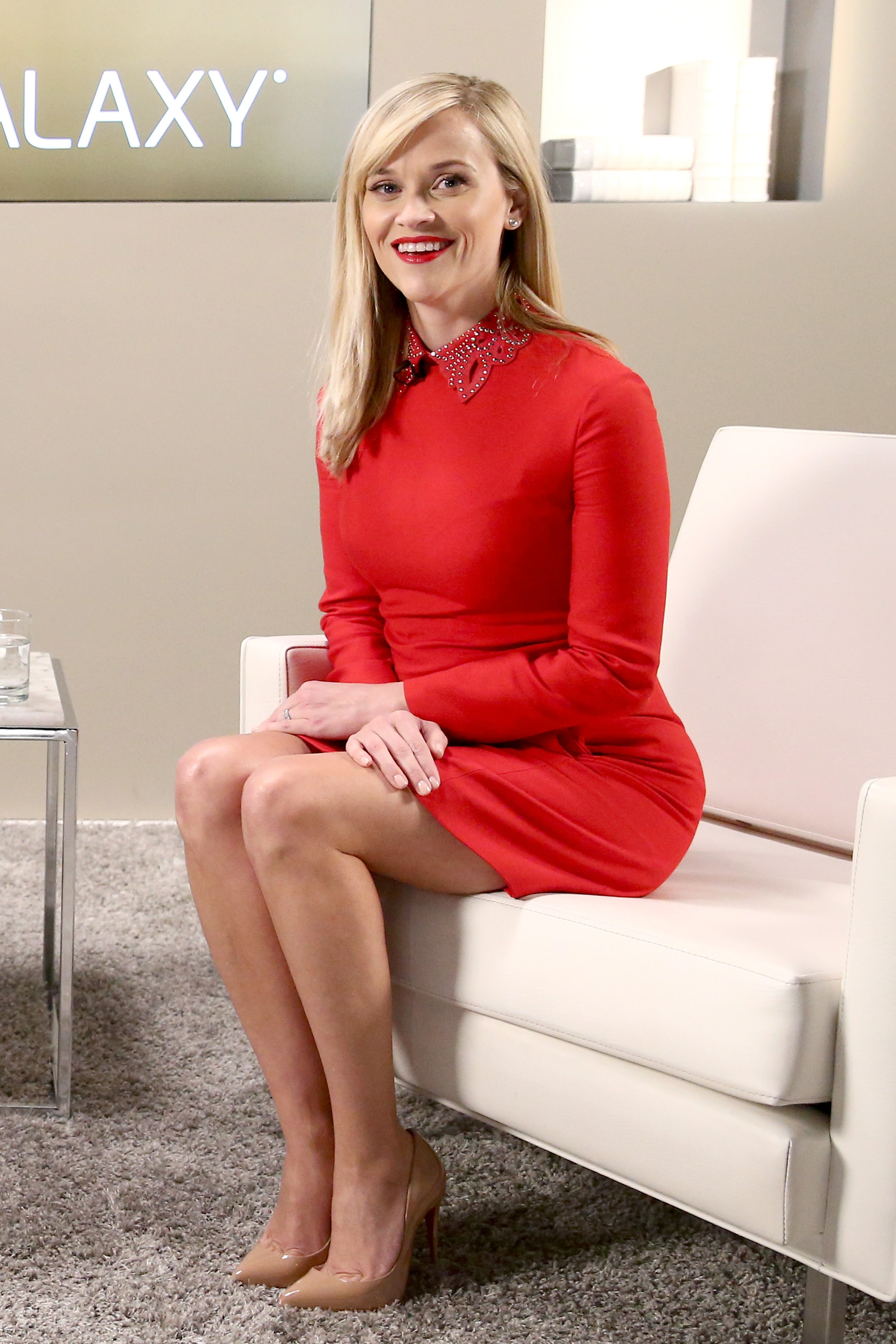The image depicts a woman who closely resembles Reese Witherspoon. She is seated on a light beige-colored sofa or chair, with her hands crossed. The woman has blonde hair parted to the side and is wearing a bright red shirt dress paired with brown peep-toe heels. Her makeup is minimal, highlighted by striking red lipstick. The dress features different silver floral patterns, particularly around the collar area. To her left, there is a side stool with a glass of water placed on it. Behind her, part of a word in white letters is visible, reading "laxy," suggesting the complete word might be "Galaxy." The background of the image is a tan color, and the carpeting has a grayish-tan hue. The photo is taken as a close-up vertical shot, and its orientation is rectangular.